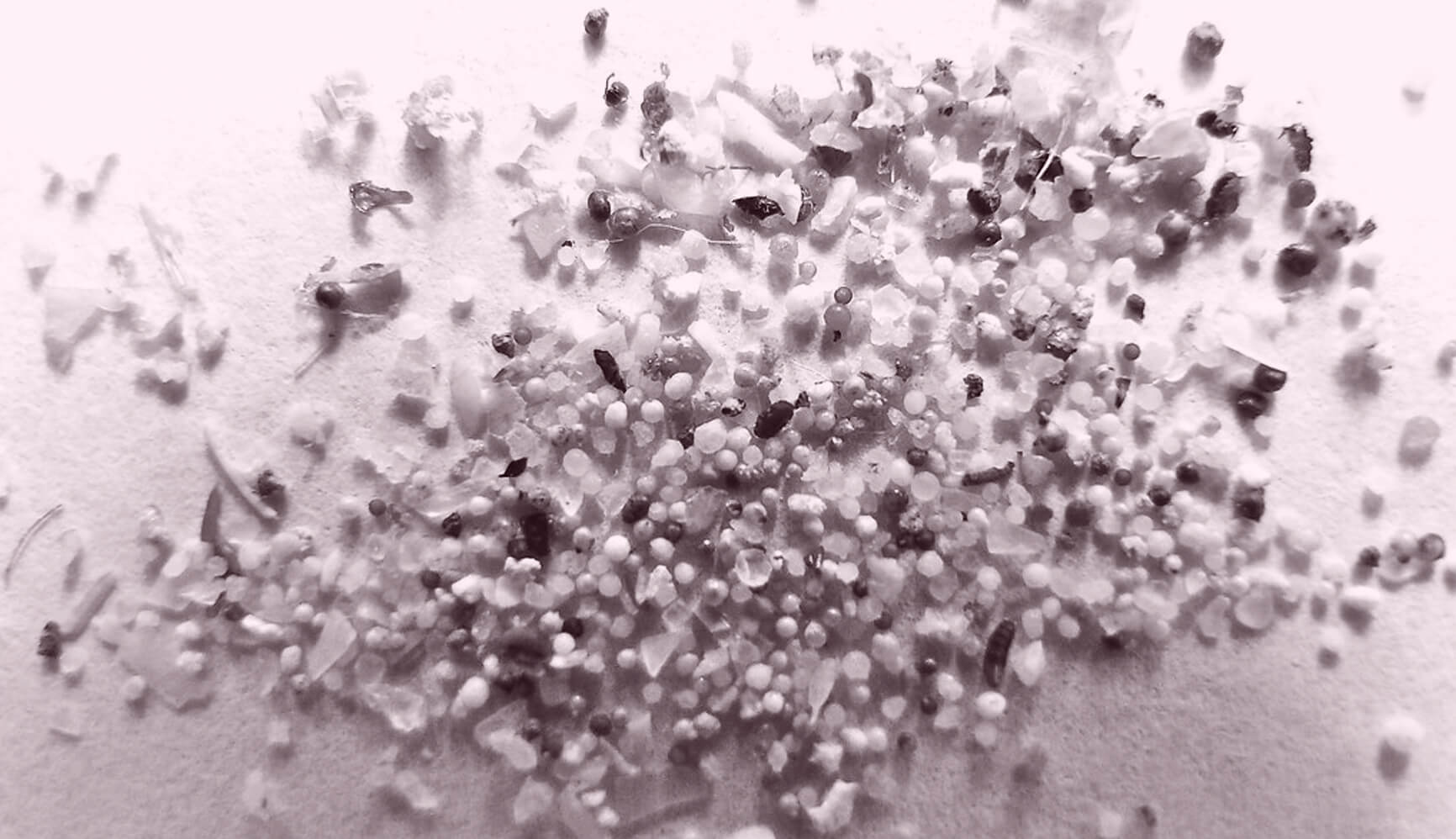This is a monochromatic, black-and-white photograph with a pinkish gray hue. The image is a close-up of small round and irregularly shaped objects scattered on a surface that appears light but is tinted with the same hue. The objects are primarily tiny beads or pebbles, varying in color from very dark to nearly white, along with a few darker, flaky elements. These elements cover almost the entire rectangular frame, with a sparser distribution on the left end. The photograph gives the impression of something that has been scattered haphazardly, possibly on a tabletop. It captures the intricate textures and varying shapes of the objects, with some being spherical and others having sharp, angular edges.